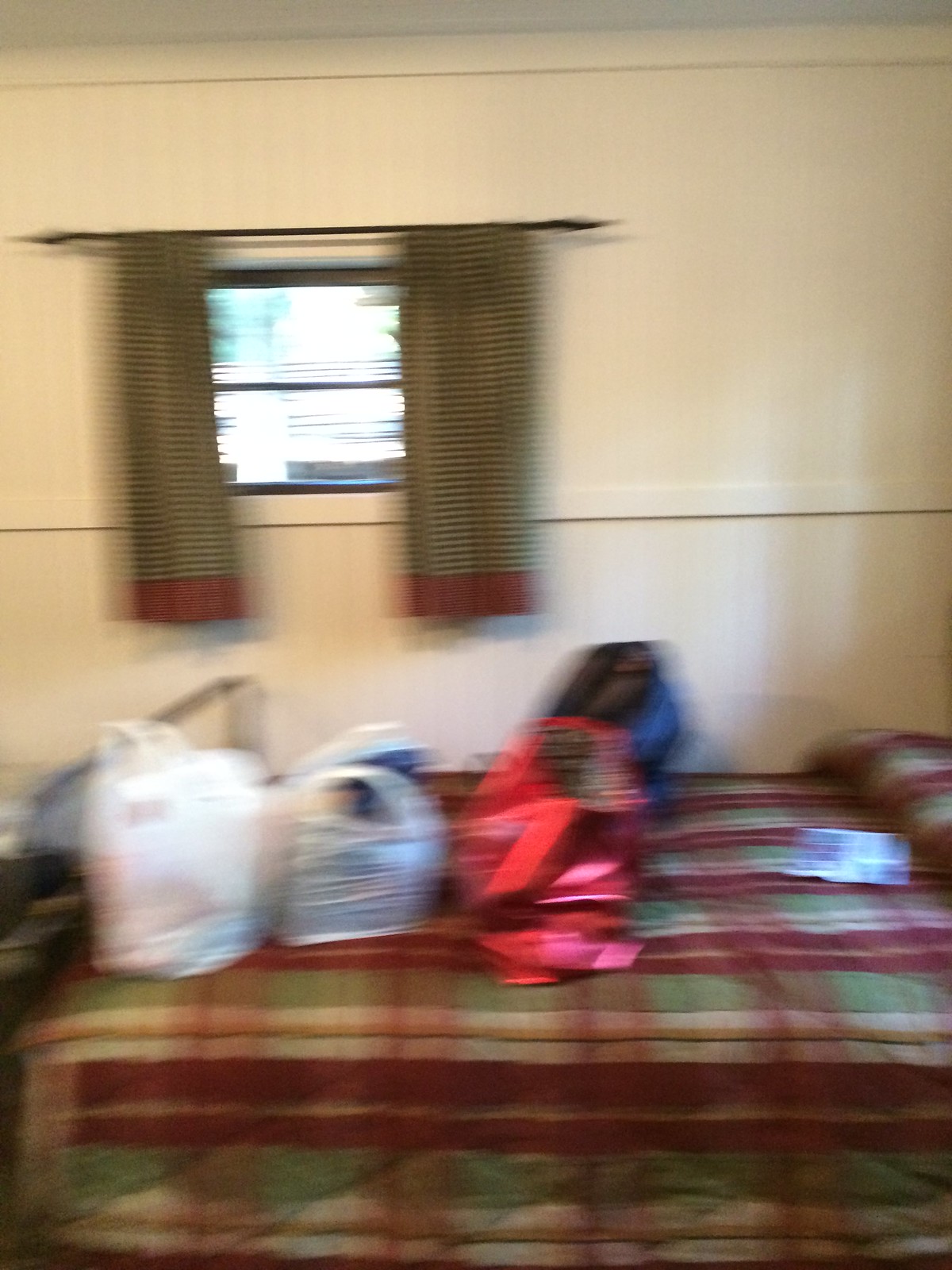The photograph, taken indoors, depicts a slightly chaotic bedroom scene captured with a shaky hand, resulting in a very blurry image. The room's white walls and ceiling provide a neutral backdrop, contrasting with the bright light streaming through a small window. The window, surrounded by a dark border, is adorned with green and black striped curtains featuring some red stripes at the bottom, all hanging from a dark metal rod. Below the window, on the red, green, white, and yellow checkered comforter of the bed, lie various items, including plastic bags in red and white, scattered haphazardly. Additionally, there are a few miscellaneous objects, potentially paper-based items like a book or magazine, adding to the cluttered yet homey atmosphere.